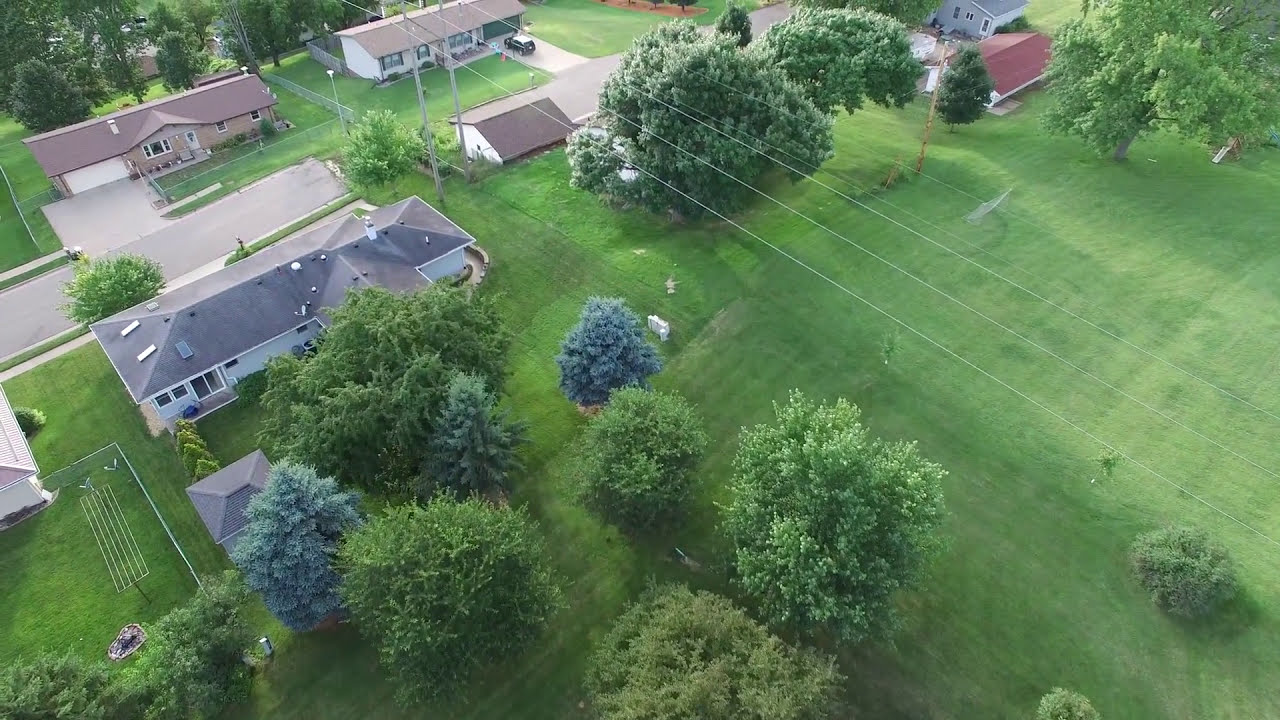This detailed aerial view at about a 45-degree angle captures a serene suburban residential area. At the upper left corner and extending off to the top right, you can see a paved road lined with houses on either side. The scene includes around six or seven distinct homes, each with meticulously maintained lawns and some adorned with large, bubbly green trees. The well-mowed grassy areas create a lush, smooth green canvas across the landscape, specifically prominent on the right side of the image, where an open expanse of green dominates. Among the visible homes, one stands out with a gray roof and white walls, while nearby, there's a beige house, accompanied by a few smaller homes. Notably, power lines diagonally traverse the view, adding a touch of everyday suburban infrastructure. Amidst the greenery, a clear day brings sharpness and vibrant color to the scene, with an impressive level of detail evident down to a single car parked in a driveway at the top left section of the image.